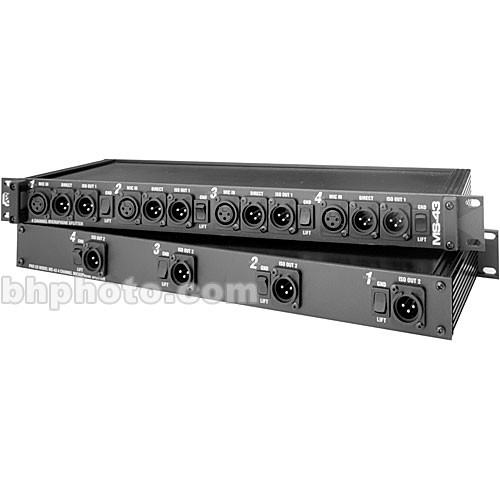This black-and-white image features two metal devices, identified as a ProSound 4-channel microphone splitter, stacked one on top of the other against a completely white background. The entire scene is monochromatic with various shades of gray. Each device appears oblong and metallic, characterized by rows of circular ports, referred to as plug prongs. The top device, marked with "MS-43" in one corner, has multiple rows of these plug prongs with tiny, barely discernible white labels adjacent to them. The bottom device is similar but features four numbered sections (1 to 4), each containing a circular port and a switch. The distinct watermark "bhphoto.com" is overlaying the bottom right corner, emphasizing the source of the image.